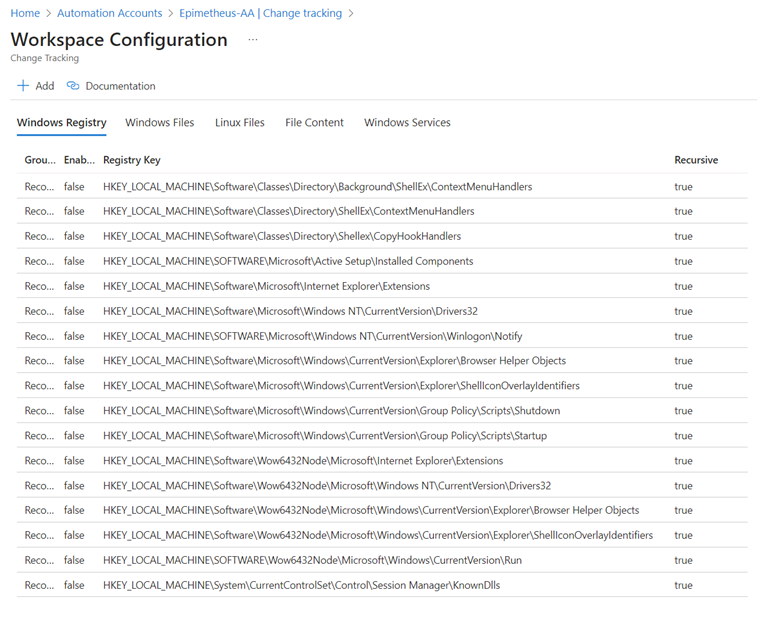A screenshot of a webpage with a clean white background predominantly featuring gray text. At the very top left, in bright blue text, it reads "Home, Automation Accounts, Epimetheus-AA, Change Tracking." This is the only text in bright blue on the page. Just below that, in gray text, is the heading "Workspace Configuration," followed by a subtitle in smaller gray text stating "Change Tracking." Further down, there is a plus sign to add items and an icon representing documentation next to it. Horizontally across the page from left to right, there are labels: "Windows Registry," "Windows Files," "Linux Files," "File Content," and "Windows Services." The "Windows Registry" label is highlighted and underlined in bright blue, indicating it is currently selected. Beneath this section is a vertical list displaying various pieces of data. The columns in this list are labeled "Group," "Enabled," "Registry Key," and "Recursive."